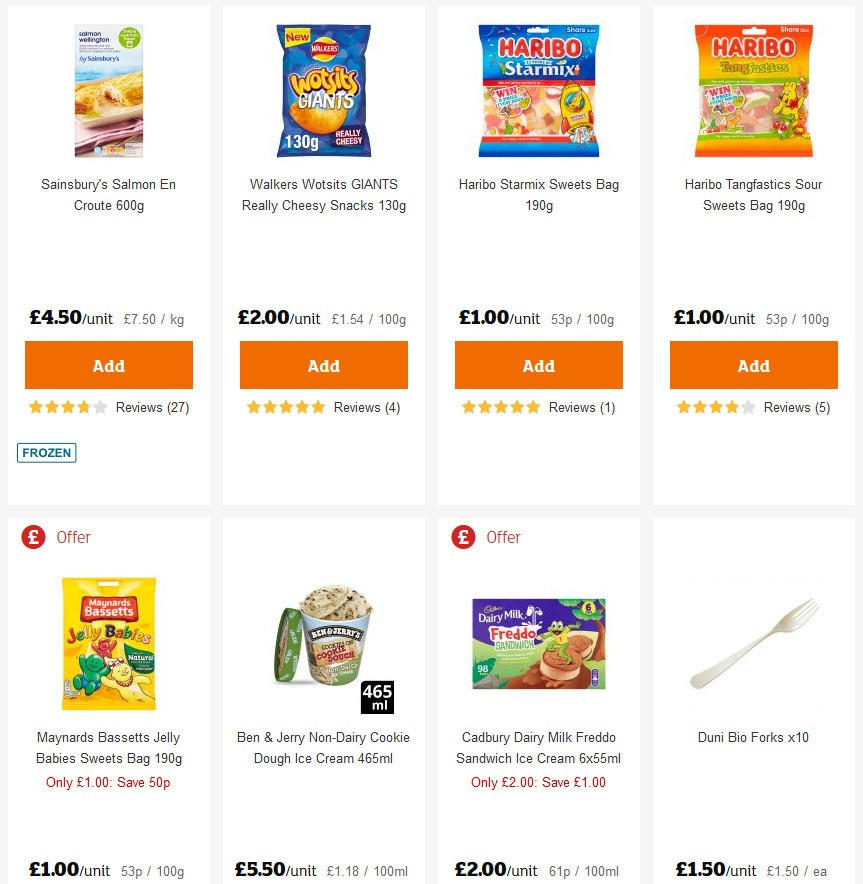The image showcases various grocery and snack items with detailed pricing, reviews, and promotional information:

1. **Sassenberry Salmon En Croute (600g)**
   - **Price:** £4.50 per unit, £7.50 per kg
   - **Features:** Grey rectangle, a white label with product picture, and pricing.
   - **Additional Info:** Four yellow stars, one grey star (27 reviews).
   - **Button:** Orange rectangle that says “Add”.
   - **Special Note:** Green outline rectangle labeled “Frozen”.
   - **Offer:** Circle with a pound sign, indicating "Offer".

2. **Walkers Watsons Giants Really Cheesy Snacks (130g)**
   - **Price:** £2.00 per unit, £1.54 per 100g
   - **Features:** Image of a bag of chips.
   - **Additional Info:** Five yellow circles.
   - **Button:** Orange rectangle that says “Add”.
   - **Reviews:** Four reviews in parentheses.

3. **Haribo Star Mix Sweet Bag (190g)**
   - **Price:** £1.00 per unit, 53p per 100g
   - **Features:** Image of a candy bag.
   - **Additional Info:** Five gold stars.
   - **Button:** Orange rectangle that says “Add”.

4. **Haribo Tangfastic Sour Sweets Bag (190g)**
   - **Price:** £1.00 per unit, 53p per 100g
   - **Features:** Image of another candy bag.
   - **Additional Info:** Four lit-up stars (five reviews in parentheses).
   - **Button:** Orange rectangle that says “Add”.

5. **Man Yard's Bessette's Jelly Baby Sweet Bag (190g)**
   - **Price:** Only £1.00, Save 50p
   - **Pricing:** £1.00 per unit, 53p per 100g
   - **Features:** Image of candy bag.
   - **Offer:** Circle with a pound sign indicating an “offer”.

6. **Ben and Jerry's Non-Dairy Cookie Dough Ice Cream (565ml)**
   - **Price:** £5.50 per unit, £1.18 per 100ml
   - **Features:** Image of ice cream, black square labeled 645ml.
   - **Description:** "Ben and Jerry's Non-Dairy Cookie Dough Ice Cream".

7. **Cadbury Dairy Milk Freddo Sandwich Ice Cream (6x55ml)**
   - **Price:** £2.00 only, Save £1.00
   - **Pricing:** £2.00 per unit, 61p per 100ml
   - **Features:** Image of ice cream sandwiches.

8. **Dooney Bio Forks (Pack of 10)**
   - **Price:** £1.50 per unit, £1.50 each
   - **Features:** Image of a fork.

Each product is accompanied by an "Add" button in an orange rectangle, facilitating easy additions to the shopping cart.